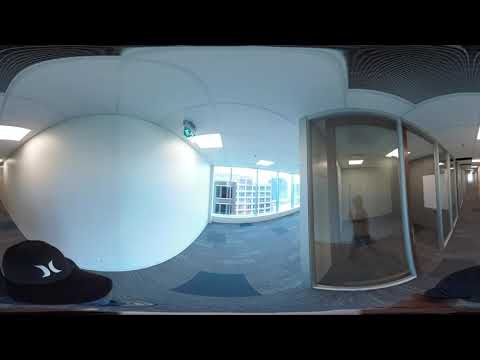The photograph, a small horizontal rectangle, captures the facade of an unusual and possibly modernist white building, set against a dark, perhaps night-time backdrop. On the left side of the image, a prominent half-circle structure—resembling a large white ball—protrudes, supported by white wooden or other similar mounting materials. Below this half-circle, in the bottom left corner, a black object, potentially the edge of a floor, adds to the scene's depth.

Centrally, expansive glass windows allow a glimpse into the building’s interior, revealing shelving units. The windows and overall design suggest the building may serve as either a business establishment or an apartment complex. To the right, the building's corridor extends, lined with more windows and cloaked in darkness, hinting at a covered walkway.

In the foreground, a black hat adorned with a logo featuring two opposing crescent moons sits prominently. Shadows and reflections, including one of a person walking, subtly animate the scene. Carpet tile floors and various shades of black, white, gray, with splashes of blue and green compose the color palette, reinforcing the enigmatic and stark ambiance of the image.